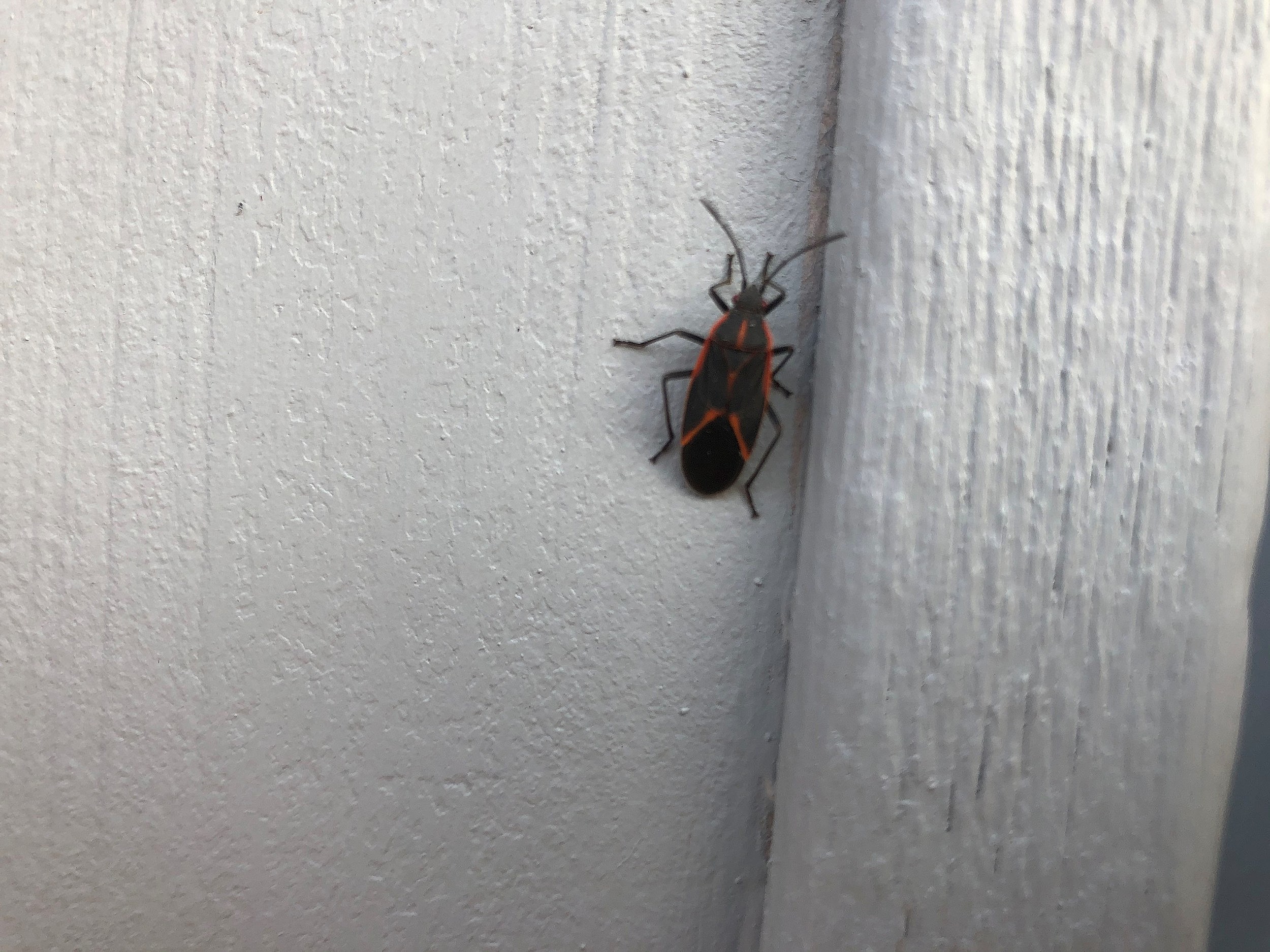The photograph features a black box elder bug prominently displayed against a white background that looks like a painted wooden wall. The background exhibits a plastery texture with a ledge or border protruding on the right side, giving the impression of some variance in the wall surface. The bug has six legs positioned distinctly: two at the front, two in the middle, and two at the back. It also has two antennae. The insect is characterized by a striking red pattern along its back, featuring two red stripes that run down its middle, with additional red marks forming a reverse V-shape near the bottom of its body. The box elder bug's wings create an oval shape, detailed with a combination of black and dark gray colors. The texture of the wooden wall and the detailed markings of the insect make this the main focus of the image.